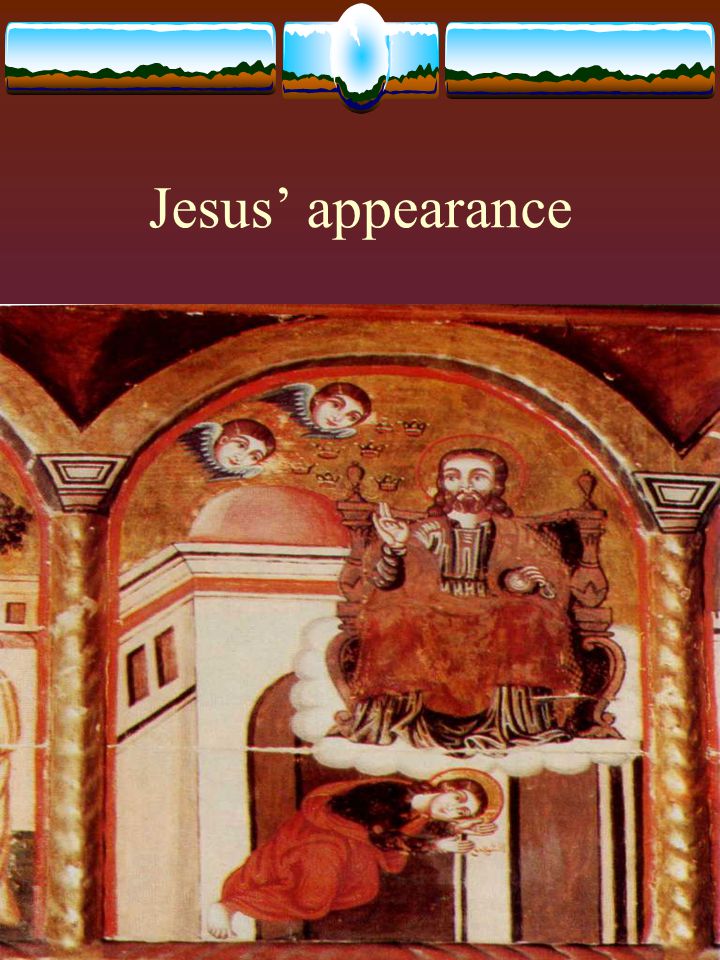At the top of this image, centered around 20% down from the top, there is off-white text against a burgundy background that reads "Jesus's Appearance." Above this text, small rectangular horizontal windows reveal a dirt terrain with distant trees and a blue sky. Below the text, the main image features a depiction of Jesus slightly off-center to the right, seated on a throne that appears to float on a cloud. Jesus is adorned in a long brown robe, with red hair, a beard, and a red halo around his head. He is raising his right hand. The scene is set within a religious building characterized by gold columns and an arched roof. Two pillars flank the image on the left and right, profiling the structure. To Jesus's upper right (the observer's upper left) is a white building with an arch and a reddish-brown dome with a couple of windows. Below Jesus, there is a woman lying down, dressed in a black shirt and a red scarf. Additionally, there are two angelic faces with wings gazing at Jesus from the left side. The floor beneath this divine tableau is covered with a red carpet. The overall impression is reminiscent of a detailed, close-up excerpt from a larger painting, stylized like a pamphlet or religious illustration.